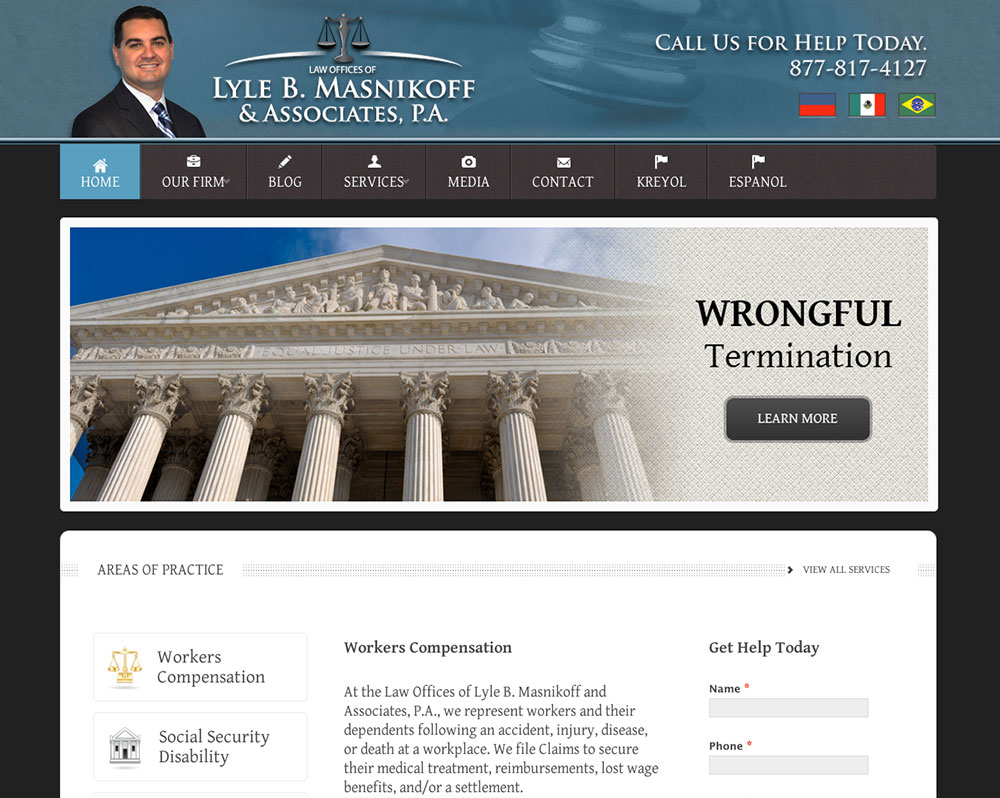The website for Lyle B. Masnikoff and Associates P.A. features a professional and user-friendly layout. At the top, a blue banner prominently displays a picture of a man alongside the text "Lyle B. Masnikoff and Associates P.A." In the top right corner, there's an invitation to "Call Us for Help Today," accompanied by a phone number. Just below this, three flags indicate multilingual support.

The main navigation menu includes categories such as Home, Our Firm, Blog, Services, Media, Contact, Creole, and Español, providing easy access to various sections of the site. A central image of a courthouse is overlaid with the text "Wrongful Termination" and a dark gray button labeled "Learn More."

Beneath, a white box titled "Areas of Practice" highlights two key service areas: Workers' Compensation with an accompanying scale icon, and Social Security Disability with a courthouse icon. To the right, a "Get Help Today" section includes text boxes for entering a name and phone number, both marked with red stars to indicate required fields.